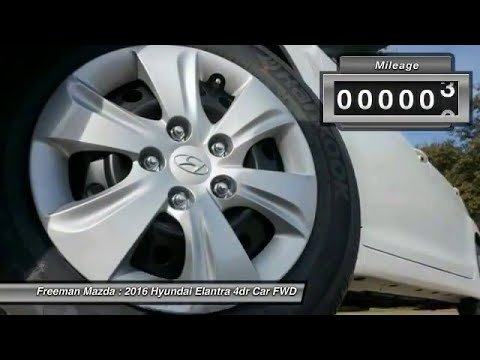The image is a close-up of the front tire of a white 2016 Hyundai Elantra. The photo, taken from the ground looking up, shows the wheel on the left-hand side, revealing the Hyundai logo in the center of the rim, surrounded by five bolts. The tire itself appears to be a Hankook brand. Positioned in the upper right-hand corner of the image, there is a gray mileage display box with white numbers, showing "00000" about to turn to "00003." Overlay text on the bottom left-hand corner reads: "Freeman Mazda, 2016 Hyundai Elantra, 4DR, FWD" against a gray background. Trees are visible in the background, but the primary focus is on the car's wheel.